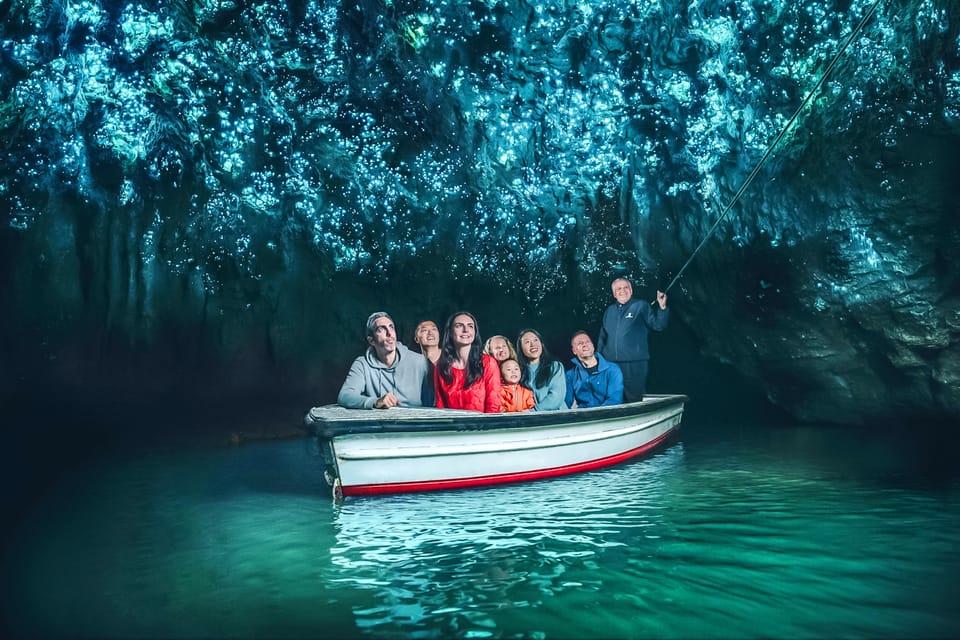This image depicts a captivating scene inside a cave where a group of eight people are seated in a boat, traversing the serene waters of a greenish-blue lake. The focal point of the photograph is the striking contrast of the boat's white and red painted exterior against the vibrant hues of the cave. An older man, positioned at the back of the boat and dressed in a black tracksuit, holds a long stick, guiding the group as they collectively gaze upwards towards the cave's ceiling. The cave's roof is adorned with glowing lights, highlighting the stalactites and stalagmites that give the cave an almost magical ambiance. The diverse group includes a man in a blue jacket with a collar, a woman in a teal long-sleeved shirt, a girl in an orange outfit, and an older woman with long hair, whose attire is obscured as she stands directly behind the girl. To their left, a woman with long black hair wears a red long-sleeved shirt, accompanied by two more men, one in a hoodie of a whitish-teal or gray color. The scene is immersive, painted in tones of blue, gray, red, and green, making the glow of the cave ceiling stand out even more against the clear blue lake, contributing to the ethereal atmosphere of this subterranean exploration.